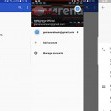This screenshot captures a small and blurry image of a computer screen displaying a pop-up menu within an application. The background features a blue banner at the top, reminiscent of the aesthetic of programs like Google Docs, possibly hinting at its origin. The entire interface is predominantly white, surrounding the pop-up. The drop-down menu, which appears to have three options, is unreadable due to the image quality. Although the text is indistinguishable, the presence of white writing towards the top alongside a blue logo—potentially Google Drive or a similar application's emblem—suggests it is a web-based tool or cloud service. The overall look implies that this is an interactive element providing a set of options to the user within the app.